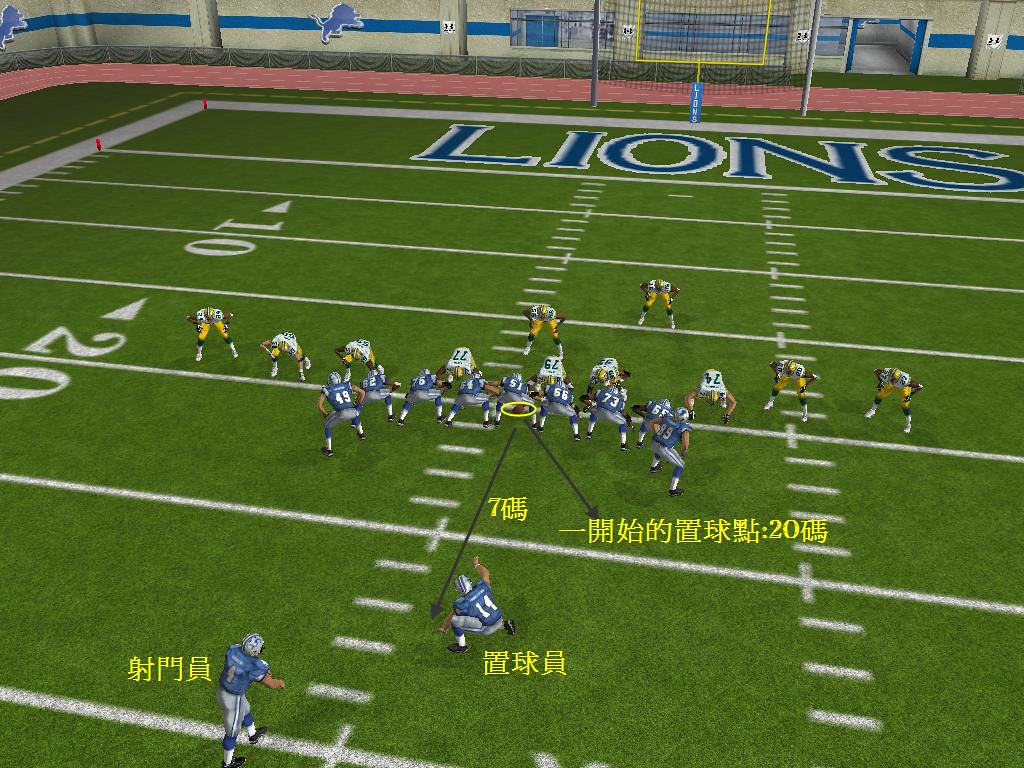The image is a detailed screenshot from a video game simulation of a football game, showcasing a moment where the blue-uniformed Lions team is about to kick a field goal. The scene focuses on the field extending to the 30-yard line, with the Lions' end zone clearly marked by the word "Lions" and adorned with a logo of a tiger or lion, backed by a wall featuring a distinctive blue stripe. The opposing team, dressed in white jerseys and gold pants, could either be the Steelers or the Rams. Visible yellow text, written in Chinese, is displayed at four distinct places on the green astroturf, adding an international flavor to the setting. The Lions players, wearing blue jerseys paired with gray pants, are strategically positioned for the field goal attempt, highlighted by two guiding lines pointing from the football towards the kicker and another line extending to the right side of the screen.